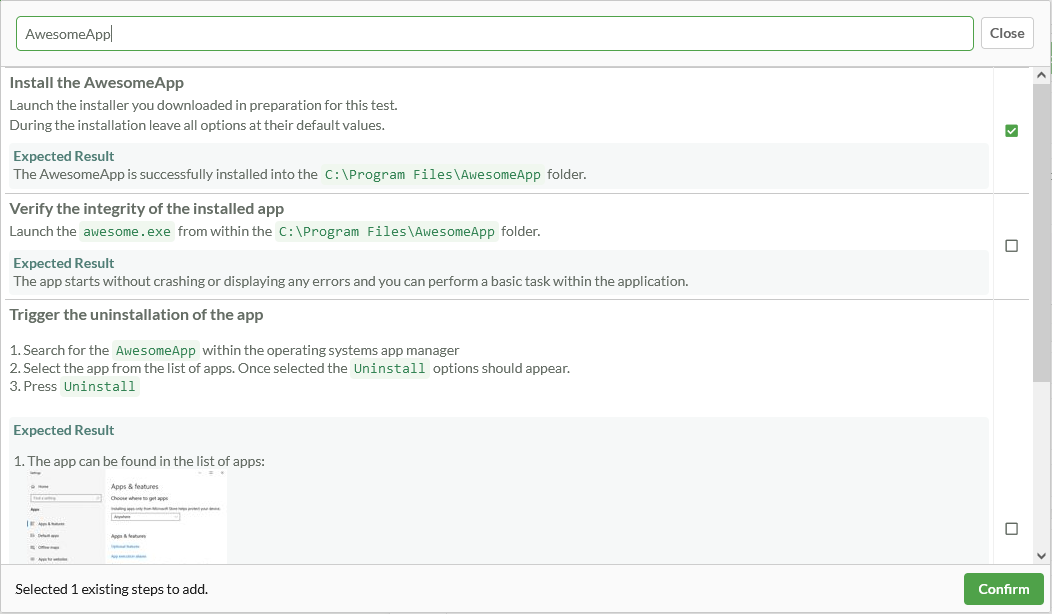This image is a computer screenshot displaying a detailed step-by-step guide for testing an application called "Awesome App." 

At the top of the picture, there is a green-outlined search bar with the text "Awesome App" typed into it. The search bar includes a gray "Close" button on the far right.

Below the search bar, several test instructions are listed:

1. **Install the Awesome App**: This instruction advises users to launch the installer downloaded in preparation for the test. During the installation process, all options should remain at their default settings. The expected outcome is that the Awesome App will be successfully installed in the C:\Program Files\Awesome App folder.

2. **Verify the integrity of the installed app**: Users are instructed to launch "Awesome X" from within the C:\Program Files\Awesome App folder. The expected result is that the app will start without crashing or displaying any errors, allowing basic tasks to be performed successfully within the application.

3. **Trigger the uninstallation of the app**: This step guides users to locate "Awesome App" within the operating system's app manager. After selecting the app from the list, an "Uninstall" option should appear. Users are then instructed to press "Uninstall."

Additionally, the image includes a screenshot of the expected result, showing where the app can be found within the system.